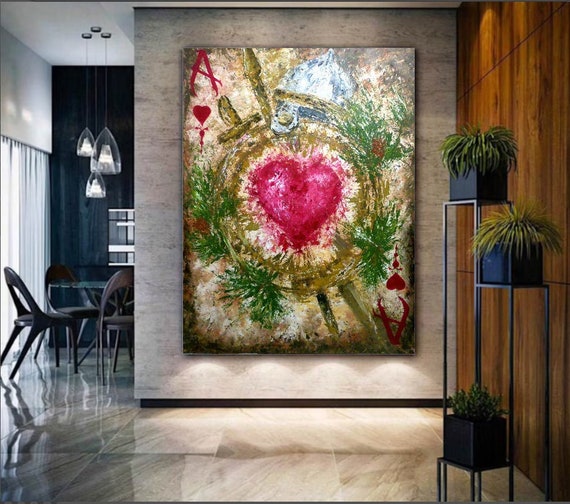This square interior photograph depicts a sophisticated and potentially upscale home setting. Dominating the center of the image is a partial stone or marble room divider, adorned with a large, abstract painting of a red heart surrounded by green decorations resembling a wreath. The painting features sketchy paint strokes, with a distinct red 'A' in the top left corner and a mirrored red design in the bottom right corner. The wall to the right is brown with dark wooden paneling, and a tiered wrought iron plant stand displays two small ferns and a succulent.

In the background, the floor transitions to light brown, highly reflective tiles that accentuate the luminescence under the painting. To the left, part of a dining set with black chairs is visible through an opening, accompanied by drawn white curtains. A glass chandelier with three triangular shades hangs above. The overall ambiance, combined with the elegant decor and marble flooring, suggests a ritzy, upper-class setting.